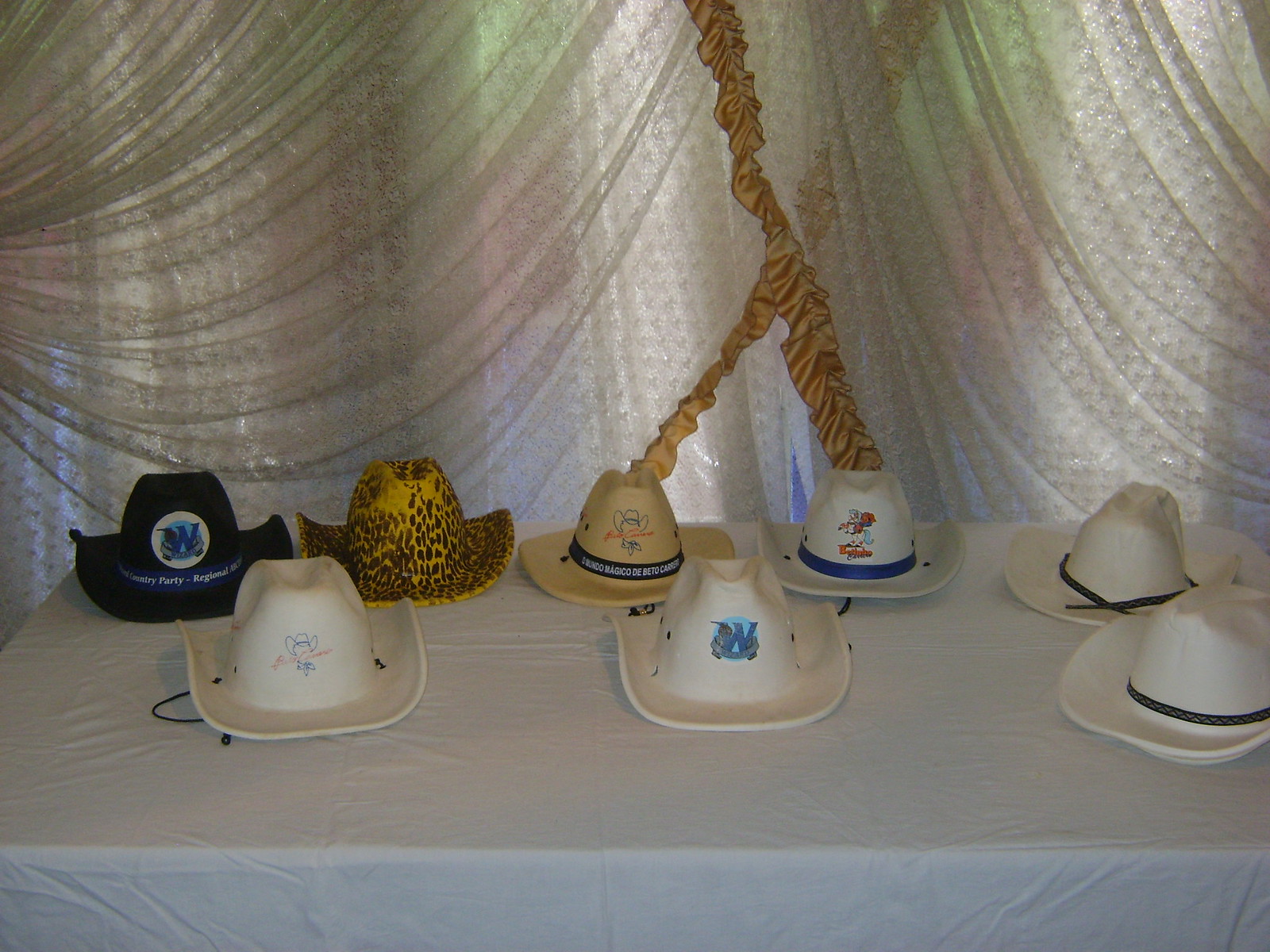The photograph captures a rectangular table adorned with a pristine white tablecloth, set against a backdrop of large, sheer white curtains with elegant tan accents and golden frills at the edges. Arranged neatly on the table are eight distinct cowboy hats. The first hat is black with a prominent white "W" in a blue circle, encircled by the words "regional" and "party" on a dark blue band. Next is a bright yellow hat dotted with dark brown polka dots. A tan hat follows, flanked by a white hat featuring a small, detailed illustration of a brown and white horse with a gray face and a blue tail. Two more white hats, each adorned with a black ribbon, sit nearby. Another white hat displays a blue circle with a dark blue "W" and a gray ribbon, accompanied by a faint bird illustration. The lineup concludes with a white hat showcasing the silhouette of a cowboy, complete with a hat, face, scarf, and red text overlaying the image.